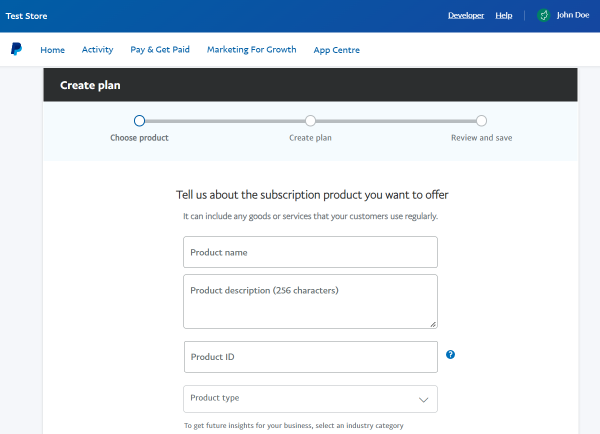This detailed screenshot captures a desktop or laptop screen displaying a section of the PayPal interface. At the top, a blue banner prominently features "Test Store" on the left and "Developer Help" on the right. Below this banner, a green button stands out next to the user name "John Doe." The PayPal logo, represented simply by a blue "P," appears prominently beneath.

The main navigation menu follows, listing sections labeled "Home," "Activity," "Pay and Get Paid," "Marketing for Growth," and "App Center." Directly beneath this navigation bar is a black banner that reads "Create Plan," aligning with the current task displayed on the screen.

Three interconnected circles with lines indicate the sequential steps in the plan creation process: "Choose Product," "Create Plan," and "Review and Save." The active step is "Choose Product."

In this section, the text prompts the user to provide details about the subscription product they wish to offer, highlighting that it can include various goods or services used regularly by customers. Four empty fields are provided for input:
1. Product Name
2. Product Description (limited to 256 characters)
3. Product ID, paired with a small blue question mark button for additional help
4. Product Type, accompanied by a dropdown arrow for selection.

At the very bottom, a prompt encourages the user to "Select an industry category to get future insights for your business."